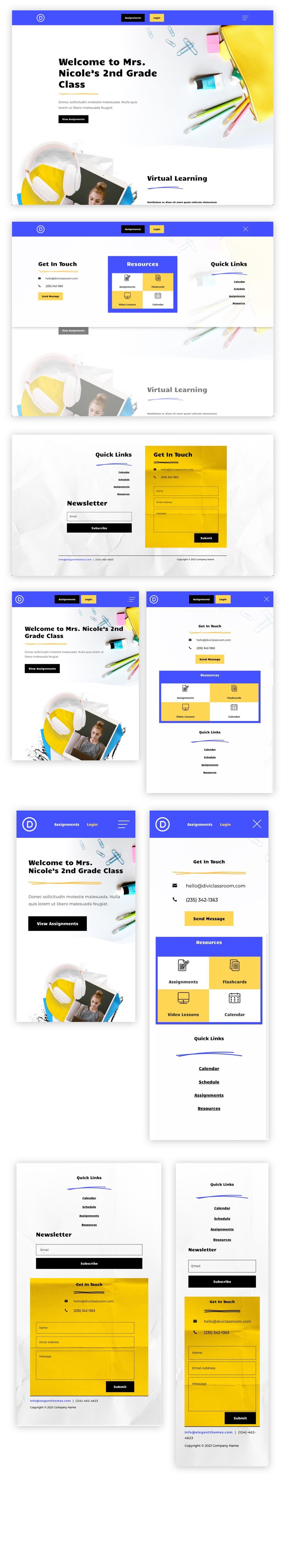The image depicts a cohesive collage of nine distinct sections, each contributing to a larger, unified visual. At the top of the composition, a long, royal blue rectangle sits above the main visual elements, providing a header. These sections collectively display the message: "Welcome to Mrs. Nicole's Second Grade Class" and mention "Virtual Learning," showcasing the digital environment for students.

The nine segments are arranged thoughtfully, with the top portion of each containing a slim royal blue header, followed by individual images against a white background. This arrangement provides a clean, organized look. The bottom of the collage features two larger boxes, each containing a prominent yellow rectangle in the center, bordered by white. These sections include quick links and a newsletter, offering accessible resources and information for the viewers. 

Overall, the image presents a welcoming and structured virtual learning space tailored for Mrs. Nicole's second-grade class, integrating both visual appeal and practical information.